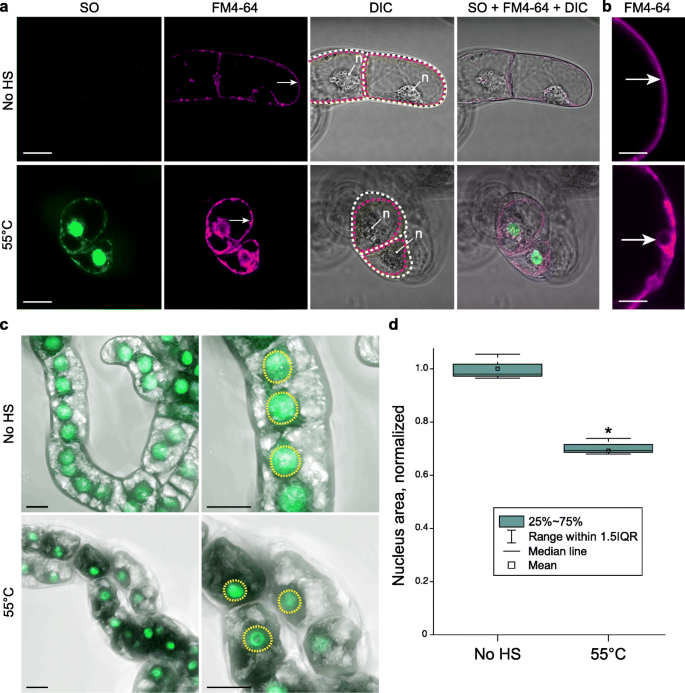The image is a detailed scientific illustration composed of numerous smaller microscope images and graphs. In the lower left corner, there are green circles moving through a clear tube, accompanied by darker images in shades of green and purple, as well as some black-and-white sections. Across the top and left sides of the image, labels such as "SO," "FM64," "DIC," and "FM4-64" are displayed. The top portion showcases cellular images, with some cells appearing gray while others are black or colored. On the bottom right, there's a line chart detailing "nucleus area normalized," ranging from zero to 1.0, with annotations indicating "no HS" on the left and "55 degrees Celsius" on the right. The chart includes a legend explaining that the range within 1.5 IQR is shown with a median line, mean, and a blue line highlighting the 25%-75% range. Additionally, white arrows and dotted lines point to specific sections of the graphs and images, providing further detail and clarity.